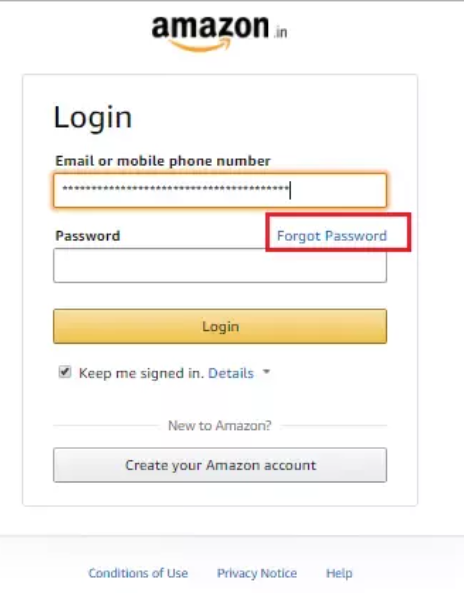The image depicts a login page on the Amazon website, characterized by its clean white background and prominent branding. At the top, the familiar Amazon logo is evident, featuring the company’s name in black with a yellow arrow underscoring it. The central focus is on the login form, where the user is actively entering their login information in a white input box accented with a yellow outline. Above the login field, the label prompts for either an email or mobile phone number.

Below this is the password field, which remains empty. A "Forgot Password" option, highlighted with a red border, is prominently displayed for easy access. Adjacent to the login fields, there is a checkbox with the instruction 'Keep me signed in’, allowing users to stay logged in for future sessions. 

A detailed description 'Details’ is provided via a blue hyperlink, presumably offering more information about the 'Keep me signed in' feature. The 'Sign-In' button below is a distinguishable yellow, signaling the action required to proceed.

Towards the bottom, the interface transitions to accommodate new users with a grayed-out prompt: "New to Amazon?" followed by a prominent rectangular button encouraging them to "Create your Amazon account." Finally, the footer includes hyperlinks for ‘Conditions of Use’, ‘Privacy Notice’, and ‘Help’, ensuring users can easily access the necessary legal and support information.